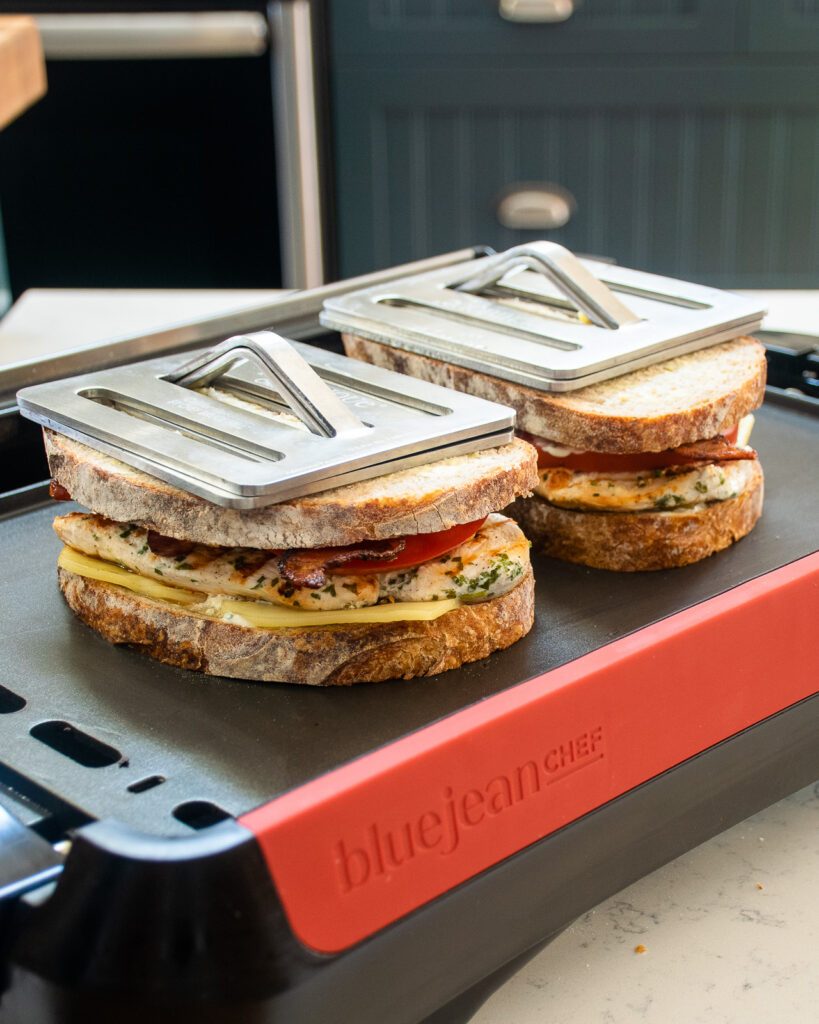The image is a close-up shot of a tabletop grill, identified as a Blue Jean Chef. The grill is black with a prominent red silicone trim where "blue jean chef" is embossed in lowercase and uppercase letters. Resting on the grill are two artisan-style sandwiches made with rustic, oval-shaped sourdough bread. The sandwiches contain various ingredients including cheese, herbed chicken, bacon, and either tomatoes or red peppers. Each sandwich is being pressed down by a stainless steel weight, featuring square forms and triangular handles with rounded tips, commonly used for ensuring even grilling. The grill is situated on a marble-effect countertop. In the blurred background, dark navy blue kitchen cabinets with vertical indentations and silver rounded handles are visible on the right side. Additionally, on the left side of the image, there is a silver vertical pole, the edge of another work surface, and a slight wooden block corner just poking into the frame, all contributing to a modern kitchen setting.